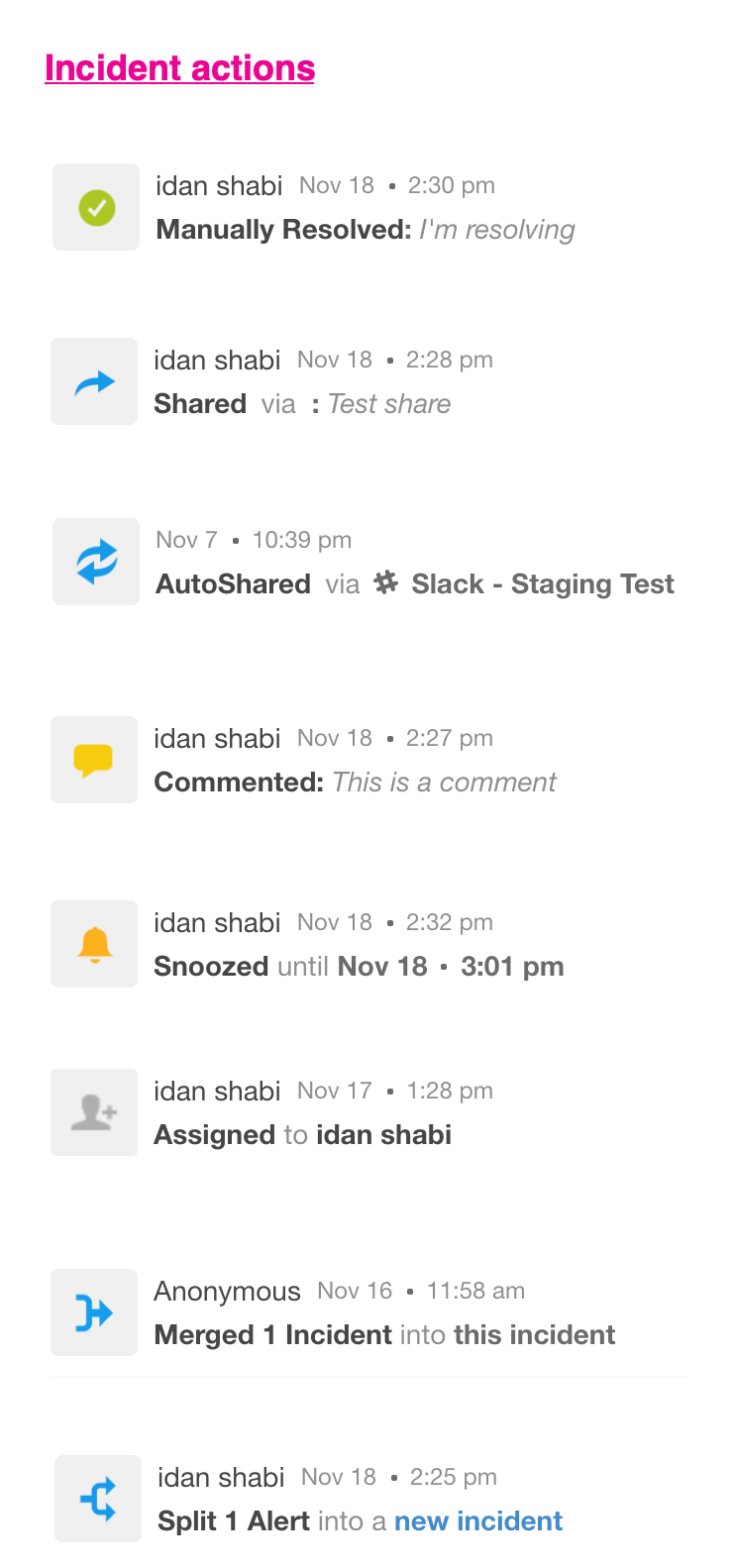This is a detailed screenshot capturing user interactions within a mobile app, displayed against a clean, white background. Centered at the top, the title "Incident Actions" is prominently written in pink, underlined sans-serif text. Below this header, a chronological list of actions taken by users is presented, each accompanied by distinct icons within gray squares.

1. A green circle with a checkmark icon:
   - User: Idan Shabi
   - Date and Time: November 18, 2:30 PM
   - Action: Manually resolved
   - Comment: "I'm resolving"

2. A blue arrow pointing to the right icon:
   - User: Idan Shabi
   - Date and Time: November 18, 2:28 PM
   - Action: Shared
   - Method: Via test share

3. Icons with a blue arrow pointing left and a blue arrow pointing right:
   - Date and Time: November 7, 10:39 PM
   - Action: Auto-shared
   - Method: Via hashtag #slack-staging-test

4. A mustard yellow chat box icon:
   - User: Idan Shabi
   - Date and Time: November 18, 2:27 PM
   - Action: Commented
   - Comment: "This is a comment"

5. An orange bell icon:
   - User: Idan Shabi
   - Date and Time: November 18, 2:32 PM
   - Action: Snoozed
   - Duration: Until November 18, 3:01 PM

6. A gray silhouette of a person icon:
   - User: Idan Shabi
   - Date and Time: November 17, 1:28 PM
   - Action: Assigned
   - Assigned to: Idan Shabi

7. A blue arrow pointing to the right with a backward C-shape facing left icon:
   - User: Anonymous
   - Date and Time: November 16, 11:58 AM
   - Action: Merged one incident into this incident

This detailed chronological log provides a comprehensive view of user activities and significant actions taken within the application.